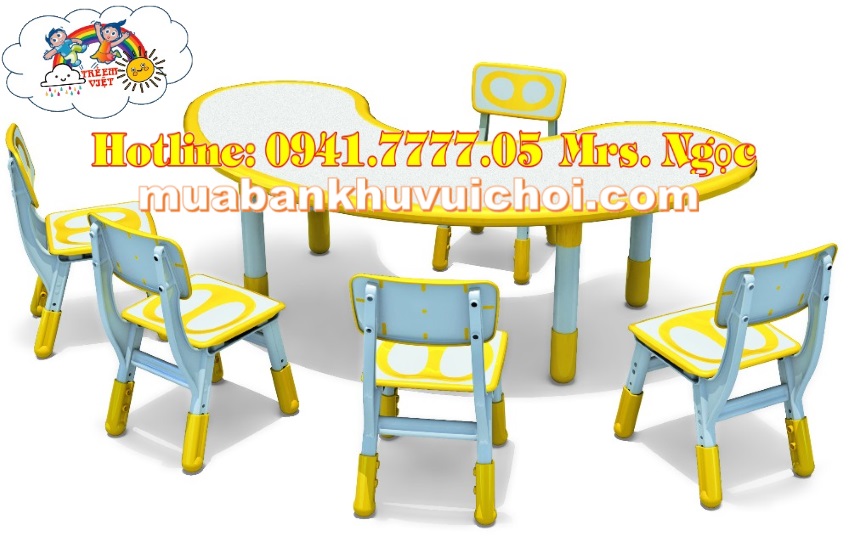The advertisement image features a whimsical, bean-shaped children's table with a white top trimmed in yellow. The table has sturdy wooden legs adorned with a bright yellow top, transitioning to turquoise in the middle, and ending with a yellow tip at the bottom. Arranged around the table are five matching chairs, each with a blue backrest that includes a playful pattern of yellow circles outlined in white and supported by yellow-tipped legs.

In the upper left corner of the image, a colorful graphic depicts a boy and a girl cartoon figure joyfully leaping in front of a rainbow. The rainbow starts from a cloud on the left end, which releases rainbow-colored drops, and ends at a smiling sun on the right. Below the children, it says "T-R-E-M V-J-E-T."

Across the center of the image, yellow text highlights a hotline number "0941.7777.05" with Mrs. NGOC's contact information. Below, it provides a web address in white letters: "MuaBankHoovachoi.com," likely directing viewers to a related website.